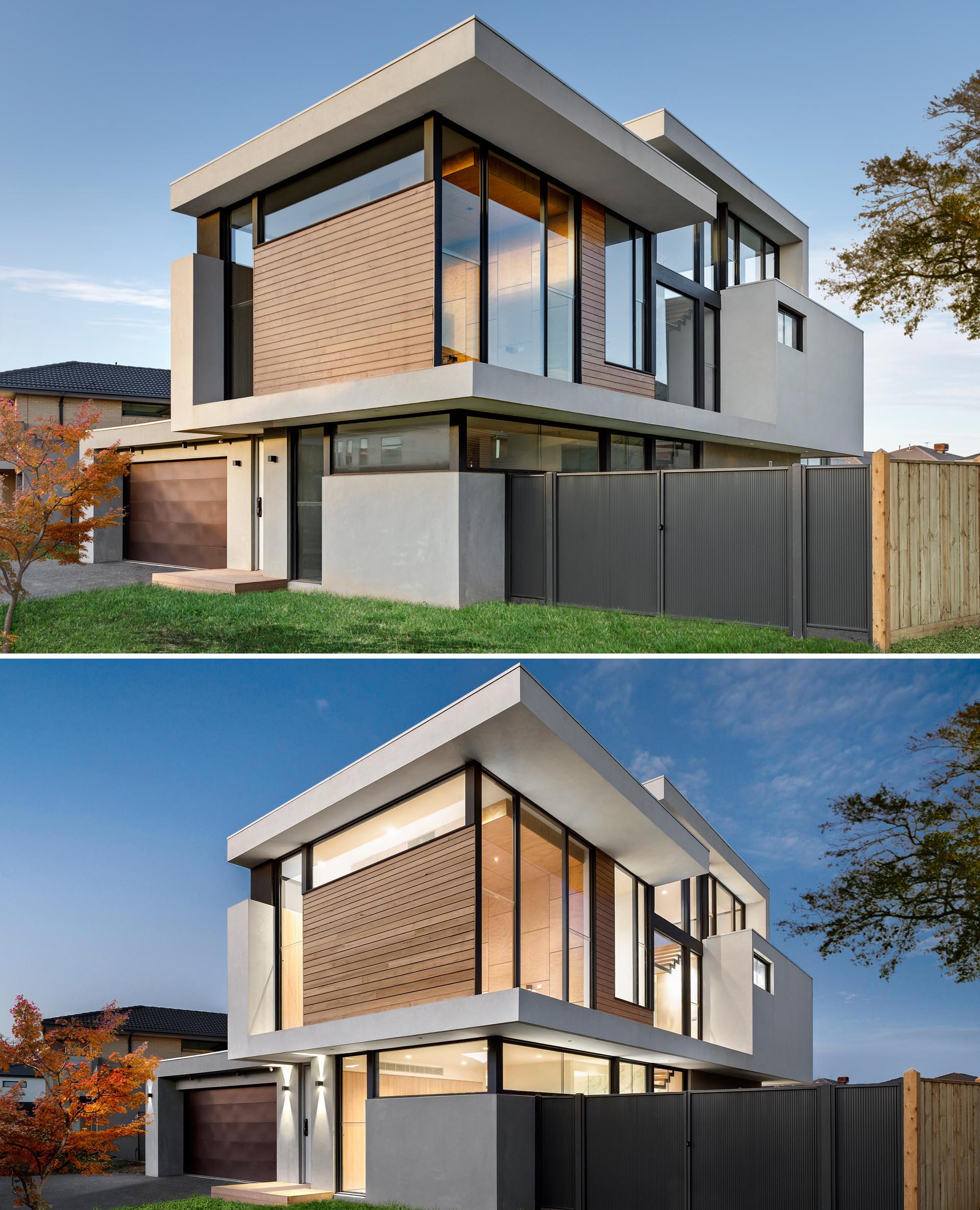This image consists of two vertically stacked photographs showcasing different times of the same modern, cubist-style house. The top photo captures the house during the day, highlighting its clean lines, large windows, and a mix of materials including gray accents and brown wood panels. The structure, featuring a garage with gray detailing, sits behind a mix of a dark-colored and light-colored wooden fence. To the right side, tree leaves peek over the fence against a backdrop of a clear, blue sky. In front of the garage, a small Japanese maple tree with reddish-orange leaves can be seen. The bottom photo, taken in the early evening with the house lights turned on, presents a slightly darker sky with faint clouds. Both images emphasize the house's modern aesthetic, abundant windows, and overall geometry, giving a comprehensive view of the exterior design from two different times of day.